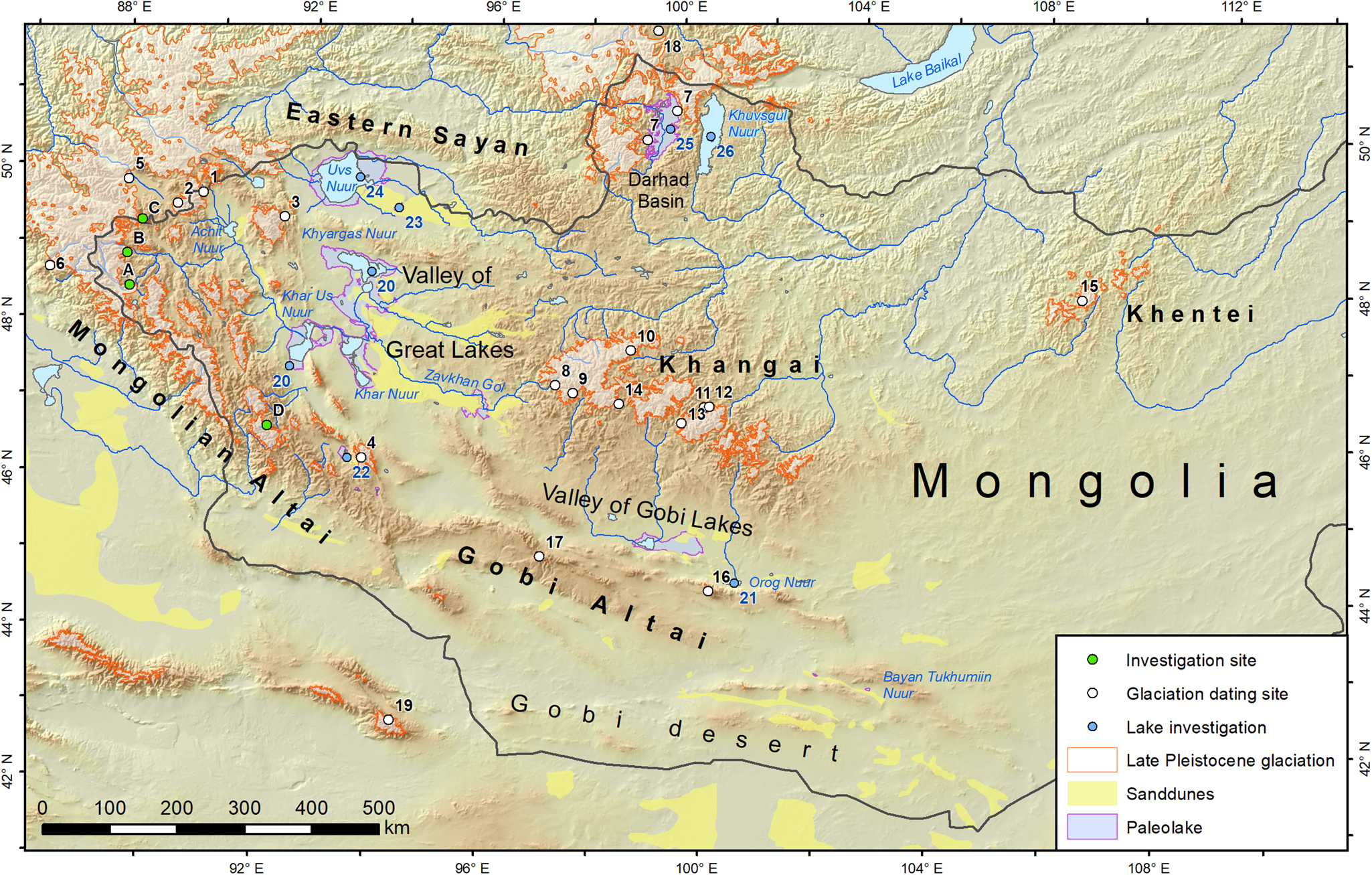This is a detailed map centered on Mongolia, displaying various key geographical features and labeled regions. The map's background is a tan color, and it includes a legend located on the right-hand side within a white square, explaining the symbols used. The legend identifies green dots as investigation sites, white dots as glaciation dating sites, blue dots as lake investigation sites, red boxes representing late Pleistocene glaciation, yellow boxes for sand dunes, and purple rectangles indicating paleo lakes.

Key regions labeled in black text on the map include Mongolia, the Gobi Desert, the Gobi Altai, the Mongolian Altai, Eastern Sayan, the Valley of the Great Lakes, and Kangai. Several rivers traverse the map, and notable bodies of water such as Lake Baikal are also shown. The map includes coordinates, with longitudinal lines marked in 4-degree increments from 88°E to 112°E, and latitudinal lines in 2-degree increments from 42°N to 50°N.

Different areas indicated by colored symbols from the legend suggest various research and geographical investigation sites scattered throughout the depicted regions, illustrating a comprehensive study of Mongolia and its surrounding landscape features.